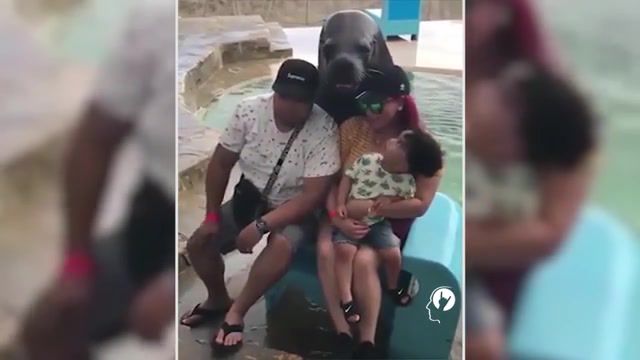The photograph captures a moment at what appears to be an aquarium or a theme park, featuring a family of three—a father, mother, and young male toddler—seated together on a blue chair. The father, situated on the left, wears a black hat, white shirt with black speckles, jean shorts, and a hot pink armband on his right arm. The mother, seated to his right with the child on her lap, sports a black and yellow striped shirt, sunglasses with a green tint, and also dons a hot pink armband. Their toddler son, who has curly brown hair, a cream-colored shirt, blue jean shorts, and black sandals, is looking up at the large sea lion behind them, which seems to be posing for the photo as well. The background features a pool of turquoise water, concrete surroundings, another blue chair, and some rock-like structures. The image, taken on a cell phone, has a blurred effect on both the left and right edges, emphasizing the clear central portion. There is a logo at the bottom right, showing a silhouette of a man’s head with a white circular hand icon inside it.